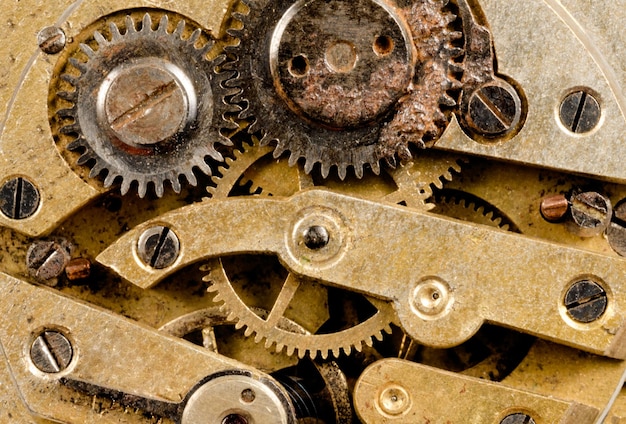This image is an up-close photograph showcasing the intricate inner workings of a machine, emphasizing a complex arrangement of gears and screws. Dominating the scene are three distinct gears—two at the top and one slightly below them. The top gears are distinctly dark, almost black, with noticeable corrosion or rust affecting their surfaces. The gear on the right features two small holes in its center, while the left one has a prominent flathead screw. Below, the arrangement reveals a prominently golden or brass gear, accentuated by oxidation and spots from wear over time. Surrounding these gears are several screws, five in total, each dark and discolored from aging. Adding to the complexity, there are golden cogs, arms, and even a spring, reminiscent of watch mechanics, although the actual machine remains unidentified. The overall color scheme includes shades of gold, brass, silver, and darkened, corroded metal, providing a vivid testament to the age and utility of these mechanical parts.